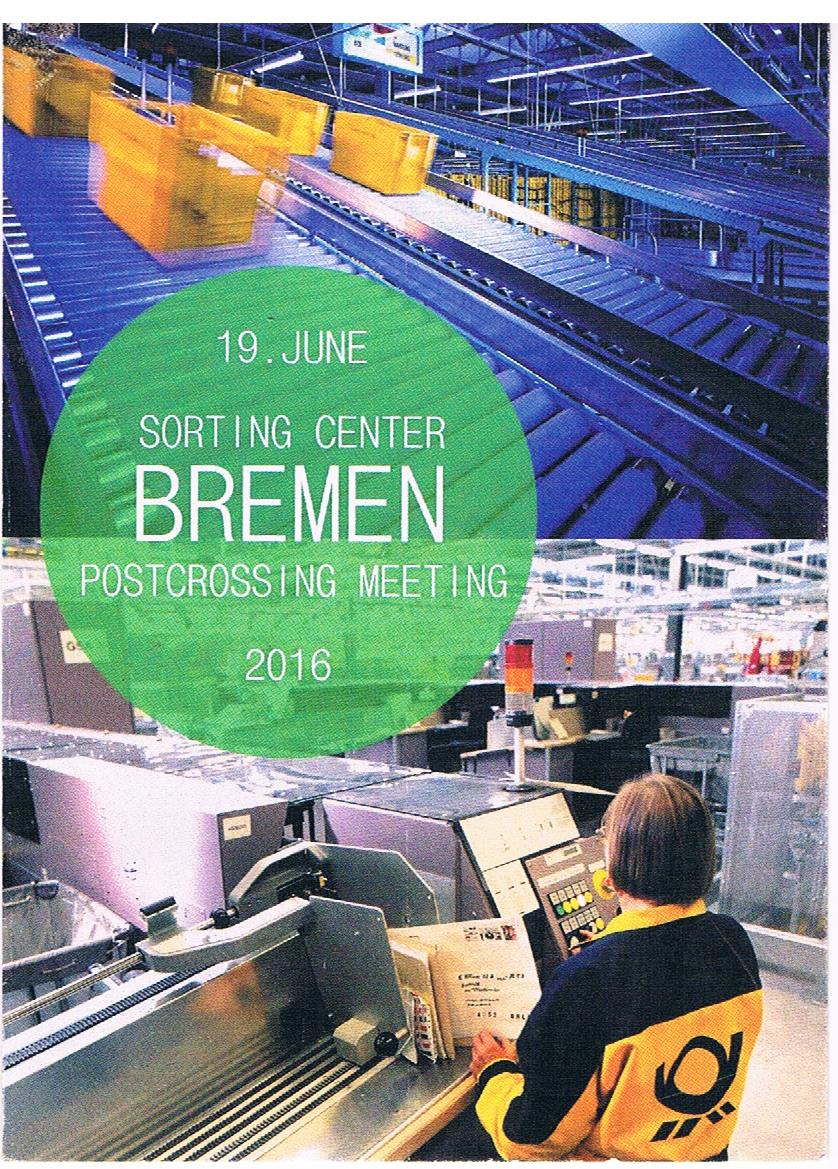The photograph depicts a busy sorting center in Bremen during a Post-Crossing Meeting on June 19, 2016. The top half of the image features a series of yellow crates moving smoothly down blue rollers, suggesting an efficient sorting system. The bottom half showcases a worker from behind, engaged with a piece of silver machinery. She is seen wearing a blue and yellow jacket, and monitoring controls with her fingers on the buttons. Her short brown bob haircut is clearly visible. Beside her, there appears to be a stack of mail. Dominating the center of the image is a large green circle, inscribed in white letters and numbers, which reads, "19 June, Sorting Center, Bremen, Post-Crossing Meeting, 2016." The entire scene is brightly lit, emphasizing the organized and active environment of the sorting center.